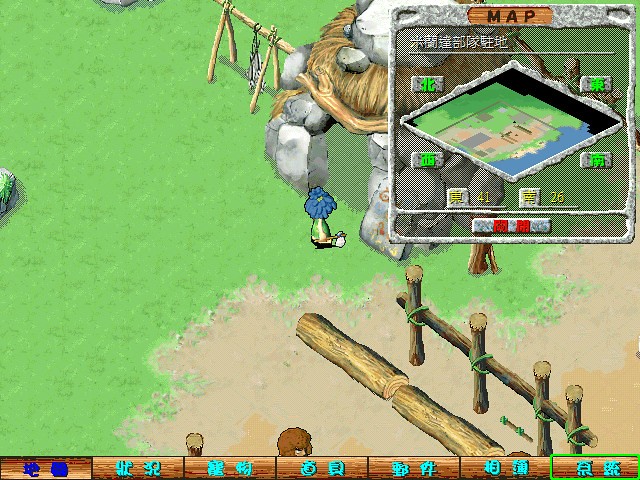This is a vibrant screenshot from a video game featuring a cartoony, child-friendly art style viewed from an isometric perspective. The scene displays text in a script resembling Asian characters, possibly Chinese. At the center, a small figure with blue hair, facing away from the viewer, holds a simple stone axe with a wooden handle. The character stands outside a quaint stone and straw hut, surrounded by various elements that evoke a prehistoric setting. Wooden logs and posts, tied together with green vines, contribute to the rustic environment. In the upper right corner of the screen, a mini map provides a localized view of the character's surroundings. At the bottom, a row of simple buttons, marked with Asian-style characters, includes one that is currently selected, indicating an active function in the game.